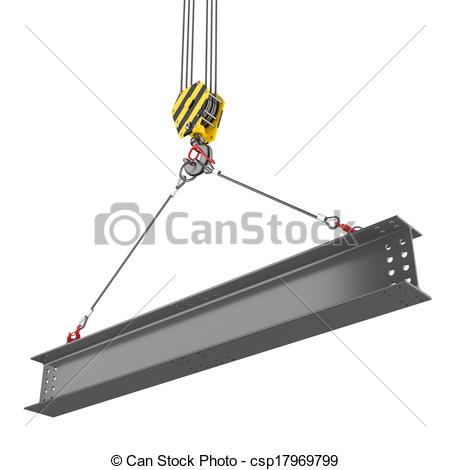The image showcases a close-up of a heavy-duty, gray steel beam being hoisted by a crane. The beam, featuring slat holes toward one end, is secured by three robust ropes, each fastened with small orange hooks. The crane's hoisting mechanism consists of a yellow and black striped metal hook or pulley system, with additional ropes attached to either end of the beam using red carabiners. The background is plain white. Overlaid on the image are stock photo watermarks, including the text "CANSTOCK" and a camera icon, with four diagonal light gray lines cutting across the scene. At the bottom, there is a copyright notice displaying "Canstock photo CSP17969799."